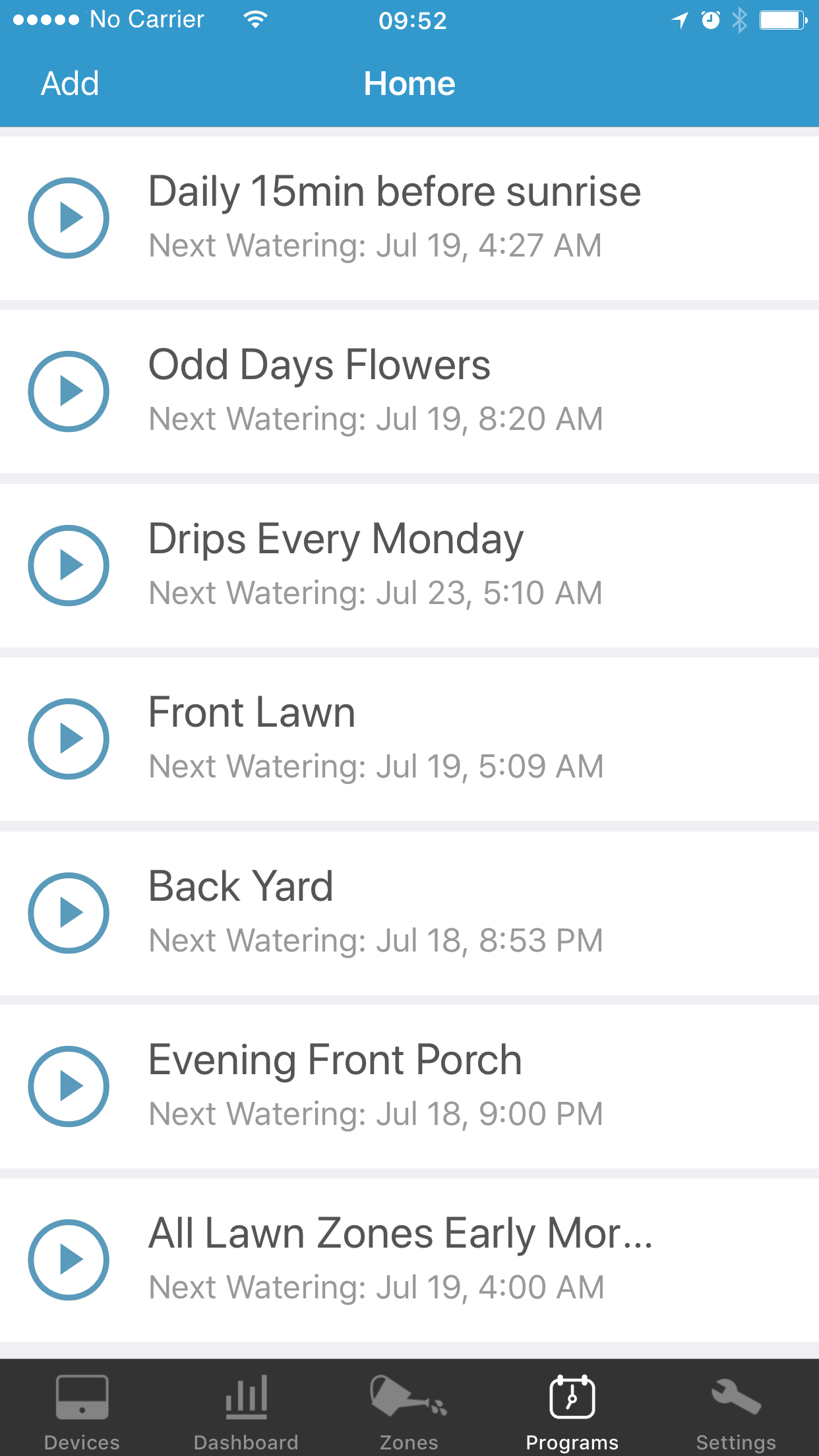This image appears to be a screenshot from a smartphone, capturing a webpage or app interface for a smart irrigation system. At the top of the screen, there is a blue rectangular header with the words "Add" and "Home" displayed in white. Above this header, the status bar shows the current time and several indicators: "No Carrier" text, a Wi-Fi signal icon, a full battery icon, a clock, and a Bluetooth emblem.

The main section of the screen displays seven rows, each containing white rectangular boxes. Each row features a blue circular play button on the left, followed by text in black and gray with different irrigation schedules. Here are the details of each row:

1. Daily 15 Minutes Before Sunrise
   - Next Watering: July 19th, 4:27 a.m. (in gray)

2. Odd Day Flowers
   - Next Watering: July 19th, 8:20 a.m. (in gray)

3. Drips Every Monday
   - Next Watering: July 23rd, 5:10 a.m. (in gray)

4. Front Lawn
   - Next Watering: July 19th, 5:09 a.m. (in gray)

5. Backyard
   - Next Watering: July 18th, 8:53 p.m. (in gray)

6. Evening Front Porch
   - Next Watering: July 18th, 9:00 p.m. (in gray)

7. All Lawn Zones Early Morning
   - Next Watering: July 19th, 4:00 a.m. (in gray)

This structured layout suggests an organized schedule for different watering zones, making it easy for users to manage and monitor their irrigation system.